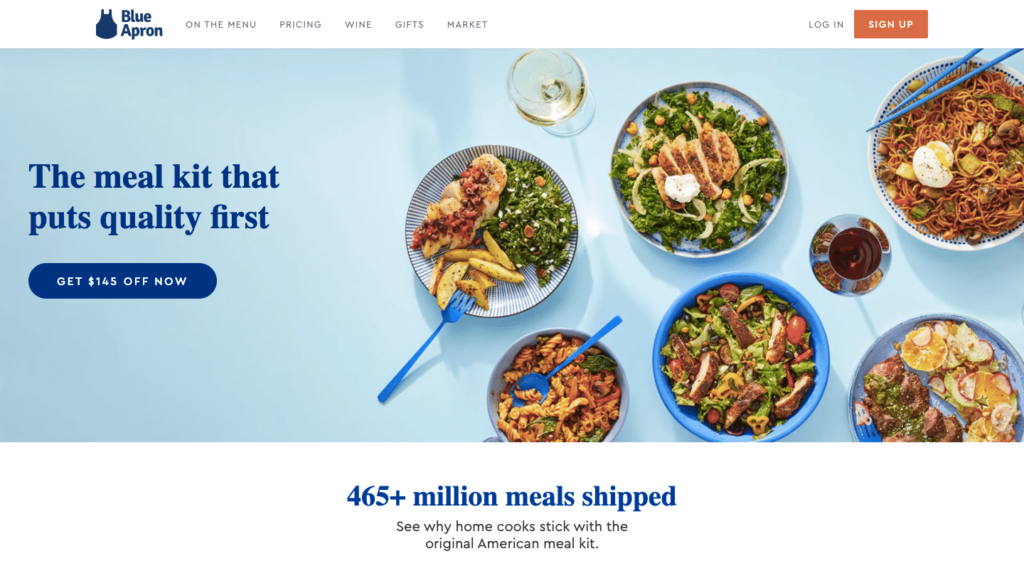The photograph captures a webpage from Blue Apron, prominently featuring a blue and white color scheme. In the top left corner, the recognizable Blue Apron logo is displayed in blue. The navigation menu at the top includes tabs for "Menu," "Pricing," "Wine," "Gifts," and "Market," accompanied by a login button. An orange sign-up button stands out against the blue banner.

Centered on the page, a bold blue message reads, "The meal kit that puts quality first," with a blue button below it urging users to "Get $145 off now." The page showcases several vibrant dishes: a wine glass filled with red wine, a blue bowl holding a colorful salad featuring chicken and tomatoes, a dish with corkscrew pasta and a blue spoon, and a blue-rimmed plate containing greens, potatoes, and fish. These vibrant images emphasize the freshness and variety of the meals offered by Blue Apron.